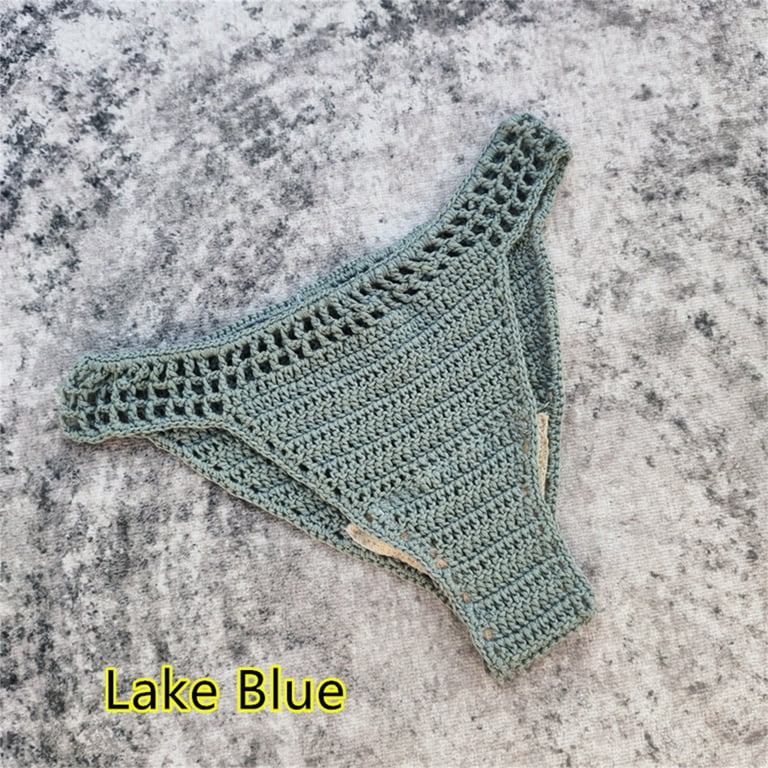The image features a knitted or crocheted bikini bottom in a light blue, turquoise, or "Lake Blue" color, prominently displayed on a gray marble countertop with black speckles. The bikini bottom showcases a unique design where the waistband has three rows of larger holes, while the rest of the garment, particularly the back and the lower section, is tightly woven. A white cloth liner is visible in the crotch area, enhancing the garment's structure. The words "Lake Blue" are written in black letters surrounded by a yellow outline, located in the bottom left corner of the image.